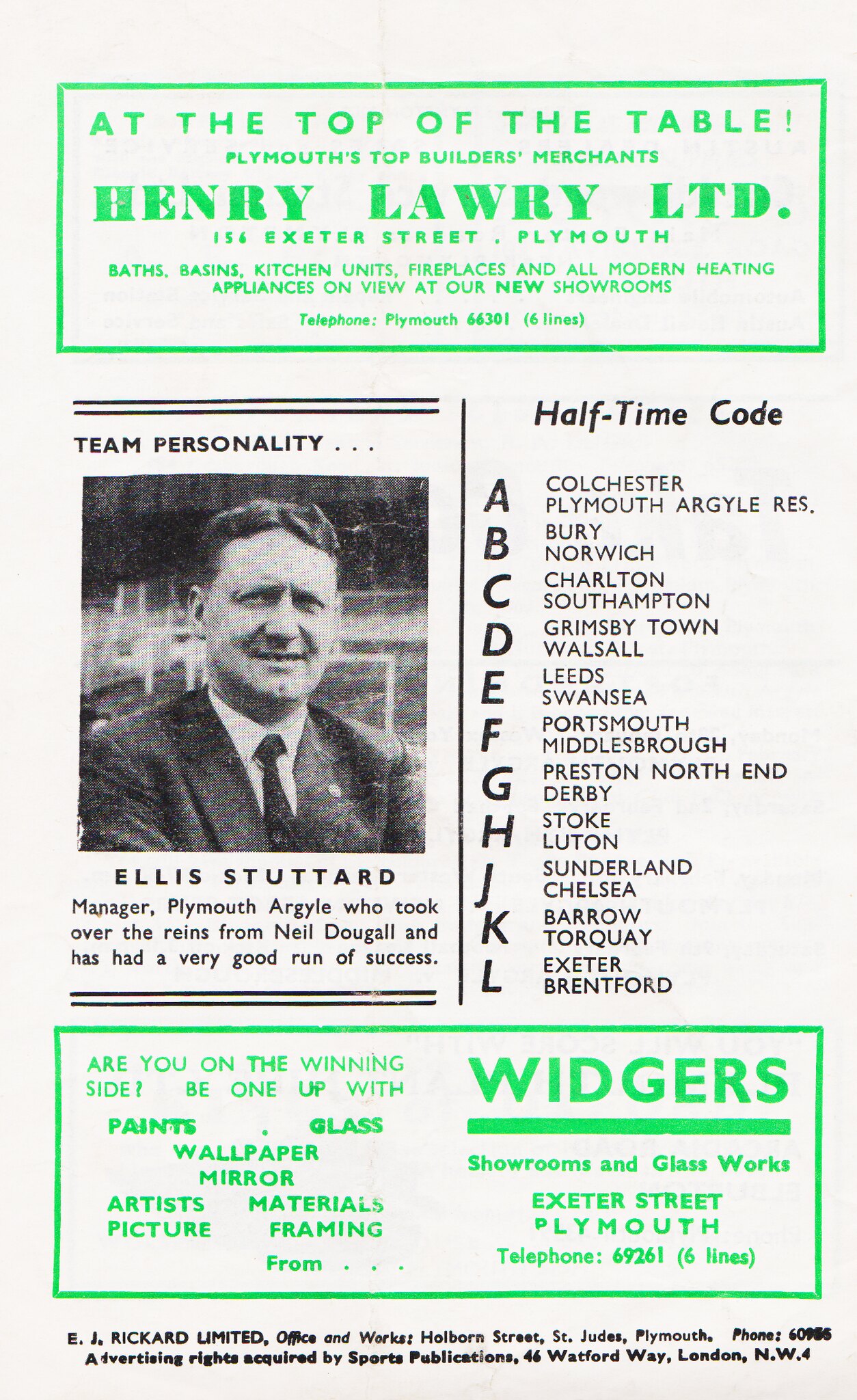This image appears to be a page from an old soccer program or newsletter, likely from the 1960s, featuring both sports content and local advertisements. The page has a white background with advertisements in a distinctive neon green print at the top and bottom. At the top, there's an ad for Plymouth's Top Builders Merchant, Henry Lowry LTD located at 156 Exeter Street, Plymouth, offering products like baths, basins, and kitchen units. At the bottom, another ad for Wink Widger's Showrooms and Glassworks on Exeter Street, Plymouth, promotes a range of items including paints, glass, wallpaper, mirrors, artists' materials, and picture framing with the catchy slogan, "Are you on the winning side? Be one up with Widger's." In the center is a black-and-white photo of Ellis Stuttard, identified as the team personality and manager of Plymouth Argyle, who succeeded Neil Dougal and has enjoyed notable success since taking the position. Adjacent to his image is a list of team pairings under the heading "Halftime Code," which includes alphabetical codes A to L (excluding I) followed by pairs of teams and cities, such as Colchester, Plymouth Argyle; Bury, Norwich; and Exeter, Brentford. The page has the aged appearance of vintage print material, slightly off-white in color, suggesting its historical context.